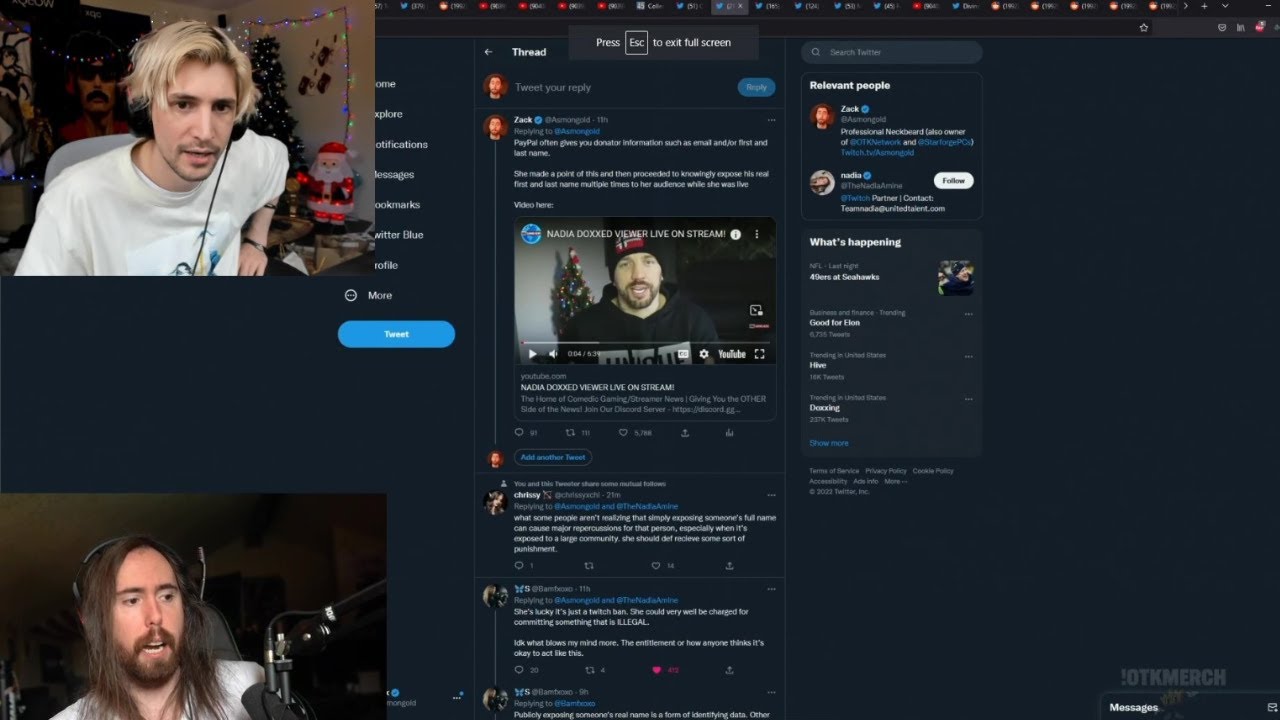This image captures a thread post featuring two streamers side by side. On the right side of the image, we see the first streamer, xQc, in the top section. He is wearing headphones and a white shirt. The background behind xQc features a Doctor Disrespect poster and some decorative Christmas lights. Below xQc, the second streamer, Asmongold, appears to be speaking into a microphone while wearing a white shirt that is slightly cut off in the image. Asmongold is also wearing gaming headphones.

On the left side of the image, the thread includes multiple posts. The first post is from Zack, identified as Asmongold, followed by a post from Chrissy. Additional posts are visible but not clearly detailed. On the right-hand side of the image, there is a "Relevant People" section that lists individuals who are pertinent to the thread discussion, and a "What's Happening" section likely highlighting trending topics or recent activities related to the content.